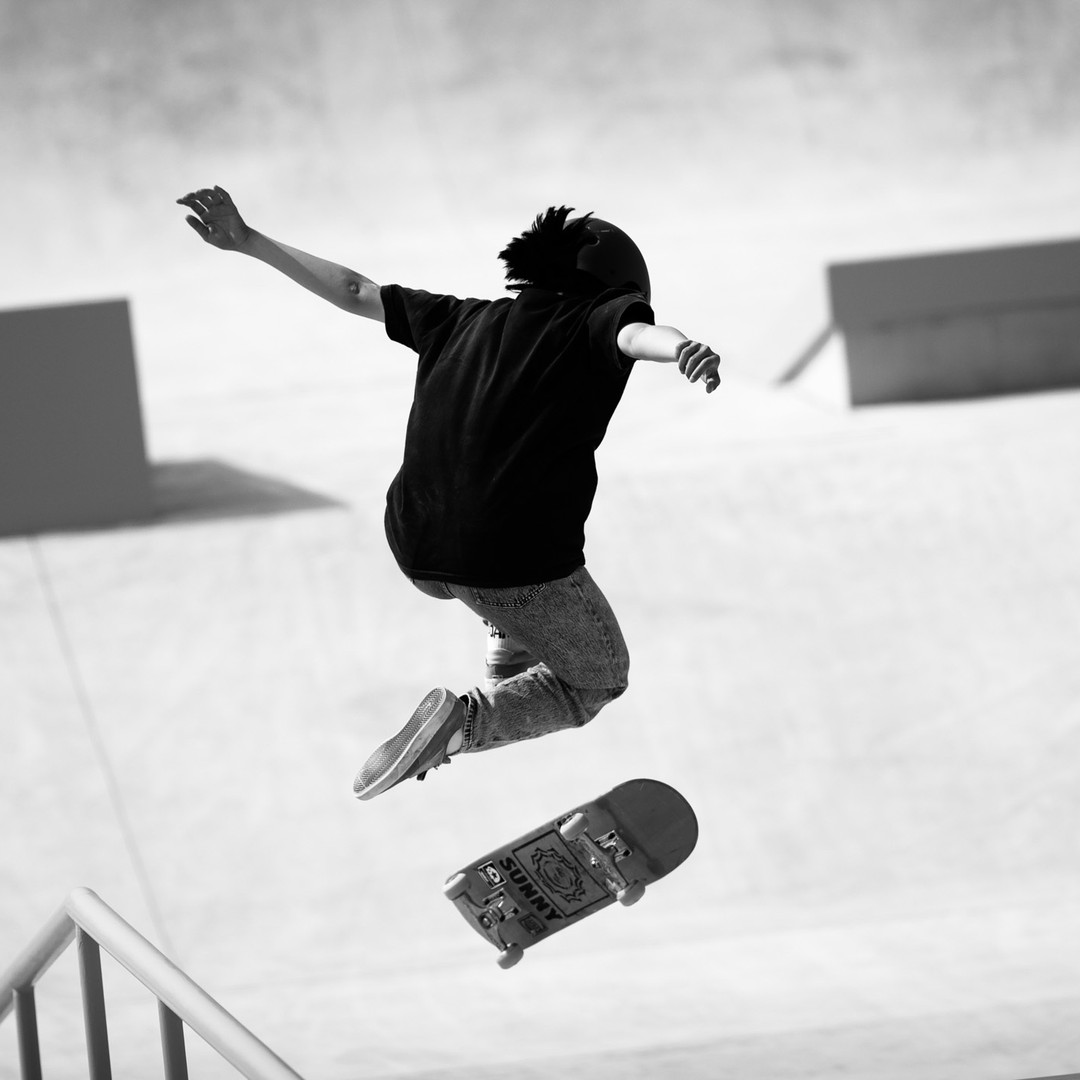In this black-and-white action shot, a man is captured mid-air while skateboarding in what appears to be a skate park. The image shows him jumping off a staircase or gap, with his skateboard hovering below his curled legs. He sports long dark hair flowing behind his head, a slightly oversized black t-shirt, and jeans, completing his skater look with flat-bottomed skate shoes. His arms are outstretched on either side, emphasizing his dynamic pose. The skateboard's underside, which features the word "SUNNY" along with a sun logo, is visible with its gray surface, white wheels, and silver trucks. The background, slightly blurred to highlight the skateboarder, includes ramps and a concrete surface typical of a skate park, along with a steel railing on the left.